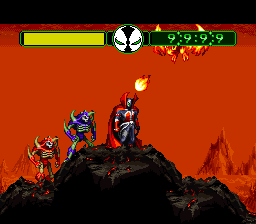This is a detailed screenshot of a video game, presented in a small square format. At the top of the image, there is a black bar. Below the bar, the majority of the background is a vivid red, depicting a fiery landscape with red hills or mountains and additional lava flows visible. In the foreground, three distinct monster-like characters are standing on a volcano-like surface, depicted with black and red lava.

The foremost monster is a striking blue, silver, and red figure wearing a red cape, with a fireball visible above his head. The second monster in the middle of the trio exhibits a blue body adorned with green spiky objects protruding from his shoulders and elbows. The final monster has a red-orange body with yellow spikes emerging from similar positions. Additionally, a fire creature is situated at the top of the image.

Overlay elements on the image include a yellow rectangular progress bar and a circle with a black, green, and white design at the top left. At the top right, there is green font displaying the numbers "9999" and a black triangle. The detailed yet small graphic composition emphasizes an action-packed and intense game environment.